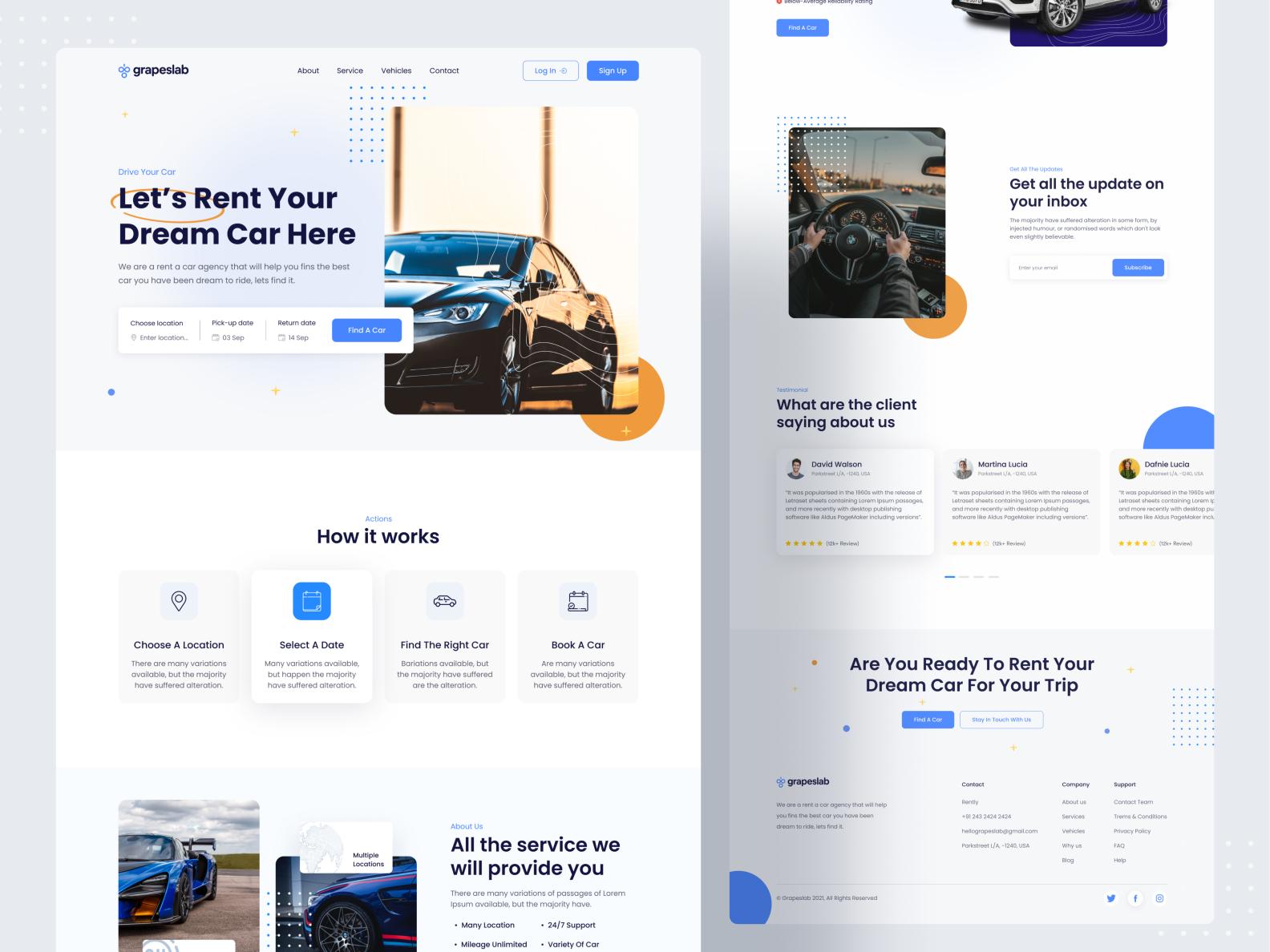**Detailed Caption:**

The website layout consists of two main sections divided into a left side and a right side, all set against a gray background. Starting from the left, there's a white rectangular area beginning about an inch in from the top left corner, extending downwards and to the center of the screen. 

In the upper left corner of this white section, the words "Grape Slab" are printed in black. Next to this text are three grape-colored circles forming an emblem. Following this, there's a list of navigation links in black: "About," "Service," "Vehicles," and "Contact," each separated by a space. 

On the right side of this section, there's a blue button labeled "Sign Up" in white text, and next to it, a white button with a blue border labeled "Log In" in black text. Beneath the "Service" and "Vehicles" links, there is a grid of blue dots arranged in 8 rows and 8 columns. 

Adjacent to this grid, in blue text, it reads "Drive Your Car," followed by a bolded black statement: "Let's Rent Your Dream Car Here." Below this tagline are two horizontal black lines. Underneath these lines is a white button labeled "Choose Location" on the left, with the instruction "Enter Location" beneath it. Further down, it displays "Pick Up Date" with "3rd of September" below, and "Return Date" with "14th of September" below that. 

To the right of these fields is a blue button with "Find Car" printed in white. Next to it, there's an image showing the side view of a black car. Beneath the image, a blue label reads "Actions," followed by black text instructing "How It Works."

At the bottom of the left section are four white buttons with blue text from left to right: "Choose a Location," "Select a Date," "Find the Right Car," and "Book a Car." Below these buttons are three lines of additional information.

At the extreme bottom left corner, there's a picture of a blue Fiero, next to another car image. Nearby, in bold black text, it says "All the Service We Will Provide You," with descriptive information underneath.

On the right side of the screen, there is more detailed information about the cars and driving experiences offered. This section includes client testimonials, and at the bottom, there is an option to plan your trip.